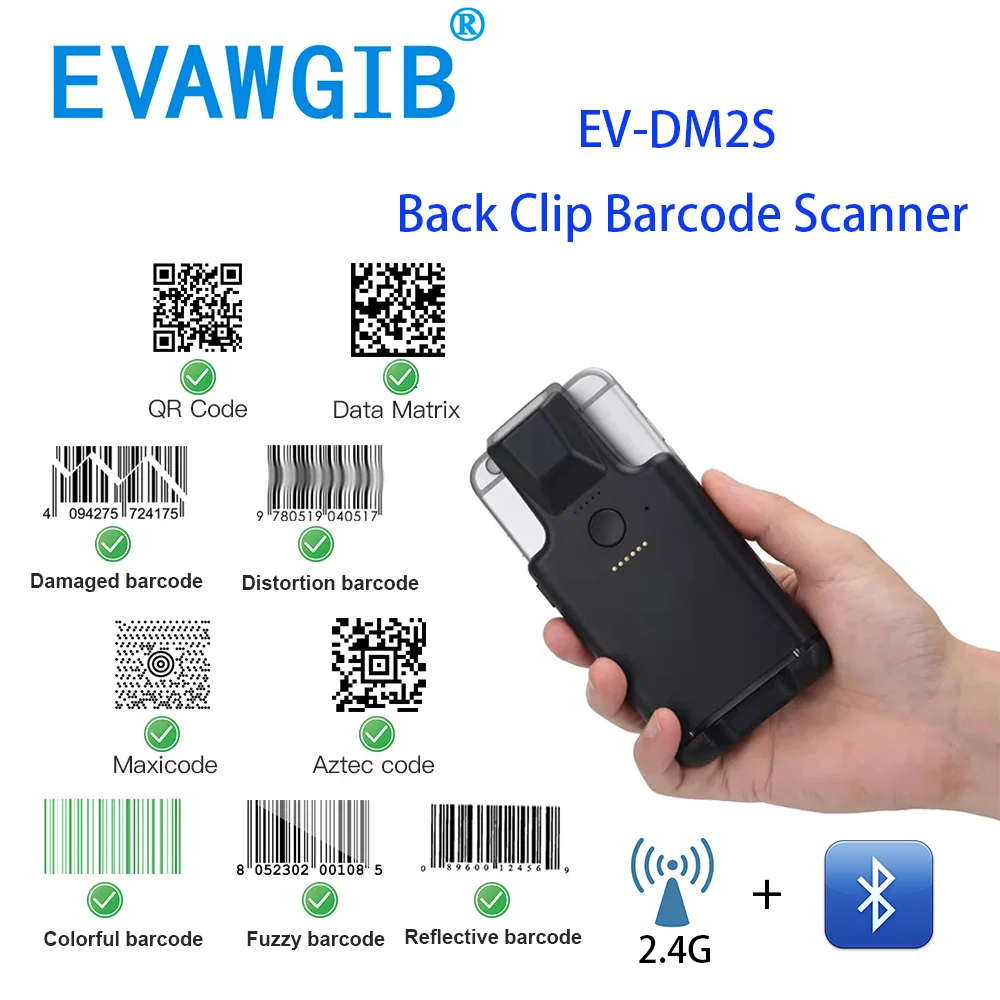The image is an advertisement for the EVAWGIB EV-DM2S BatClip Barcode Scanner, featuring a white background. The logo "EVAWGIB," in blue font with a registered trademark symbol, is located in the upper left corner. Below it, in black font, reads "EV-DM2S, BatClip Barcode Scanner." The central right portion of the image shows a white hand holding a silver smartphone, equipped with the black BatClip Barcode Scanner, which attaches around the bottom and sides of the phone with a button in the center. Down the left side, there are images showcasing the scanner’s compatibility with various barcodes, each marked with a green checkmark: QR Code, Data Matrix, Damaged Barcode, Distortion Barcode, Maxi Code, Aztec Code, Colorful Barcode, Fuzzy Barcode, and Reflective Barcode. At the bottom, a blue triangle and dot with Wi-Fi symbols and "2.4G" text is depicted, followed by a plus sign and the Bluetooth symbol in a blue square, illustrating the device's connectivity options.